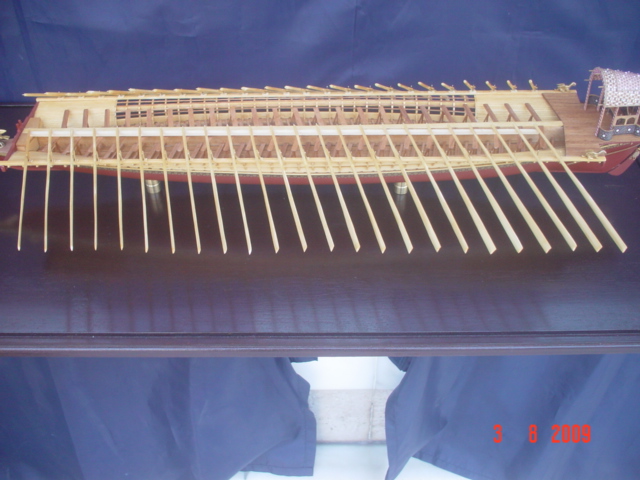This detailed caption amalgamates the shared and repetitive information from the three descriptions provided:

The image depicts a detailed model of a long, historic ship, showcasing the intricate interior and framework as though the ship were cut in half to expose the bottom half. The model highlights the craftsmanship with multiple wooden oars extending out from both sides, suggesting its use as a rowing vessel from a bygone era. The ship's reddish-brown hull contrasts with its tan deck, which includes a small covered area at the far end. The model is mounted using two small silver bolts to a flat blue surface, possibly within a glass display case. Behind the table is a blue backdrop, while the bottom of the photo reveals glimpses of a white floor below the blue surface. Notably, the lower right corner of the image bears a red date marking, "3-8-2009," indicating when the photo was taken.